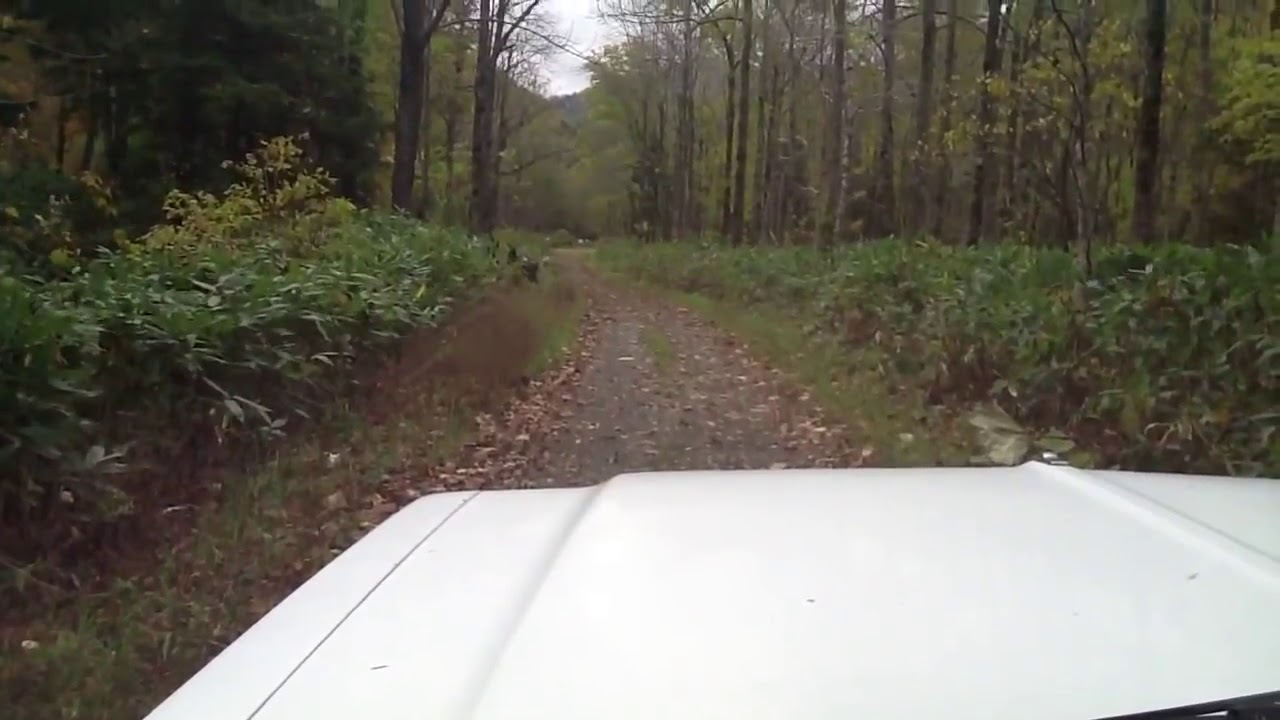This photograph captures the view from inside a white vehicle—possibly a car, SUV, or pickup truck—traveling along a narrow, brown dirt path in the middle of a dense jungle or wooded area. The bonnet of the vehicle is visible in the forefront against the uneven, unmetalled pathway scattered with dry, orange-brown leaves. Both sides of the path are densely lined with green grass, shrubs, and tall trees, creating a secluded, natural corridor enveloped in rich greenery. Overhead, the sky peeks through the canopy, appearing mostly gray and cloudy, giving the impression of a tranquil, overcast day. The jungle seems alive with mid-season foliage, providing a lush but desolate landscape surrounding the vehicle on its journey.